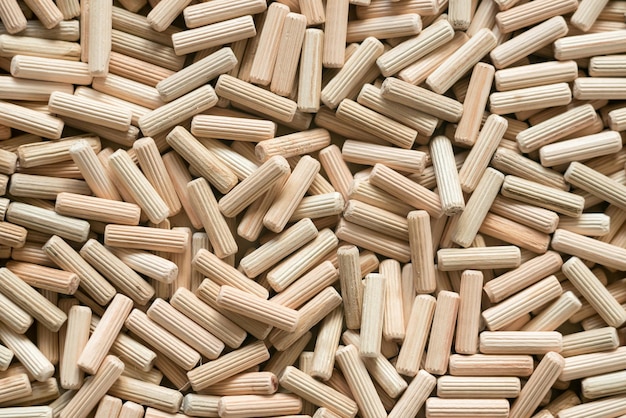This highly magnified color photograph depicts a jumbled pile of numerous small, cylindrical objects that resemble wooden dowels or pegs. These pieces are light brown to almost white in color, suggesting a varying beige palette throughout the mass. Each dowel is approximately 1.5 to 2 inches in length, featuring indented lines or ridges running vertically along their surfaces. The dowels have open ends, mimicking the appearance of tubular structures similar to pen caps or small rigatoni pasta. The image presents these dowels scattered in all directions, densely covering the entire frame with no visible background, adding to the sense of clutter and abundance. While the precise material of the dowels is unclear—potentially plastic or wood—their appearance is reminiscent of the wooden dowels commonly used in furniture assembly, such as those from IKEA, to connect two pieces of wood without screws or nails.